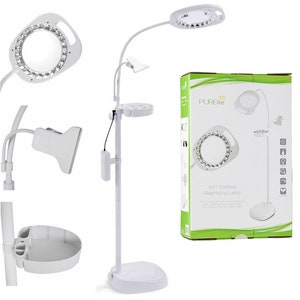This image is a screenshot showcasing a medical product available on Amazon, likely within the images tab of the product listing. The product is prominently displayed in the center of the image against a plain white background, creating a clean and professional appearance.

The central product is a dentist's light, featuring a sleek, off-white and gray finish similar to the lighting typically found in a dental office. It includes a sturdy light stand with a tray attached, housing some electronic wiring that connects to a handheld controller.

The stand itself has a circular base for stability and extends vertically with a slight curve near the top, resembling almost a right angle. Midway up the pole, there's an additional accessory attached via a black wire that appears to be used for remote control functionality.

At the apex of the pole, the light fixture is positioned to cast illumination directly downward, likely intended for use during dental procedures. The light fixture is divided into three distinct components on the left side, perhaps to allow for flexible lighting options.

Accompanying the product in the image is its packaging – a white box featuring a picture of the product on the cover. The box is accented with a green outline, adding a subtle touch of color to the otherwise monochromatic image. The box is positioned to the right of the product, providing potential buyers a glimpse of both the item and its packaging.